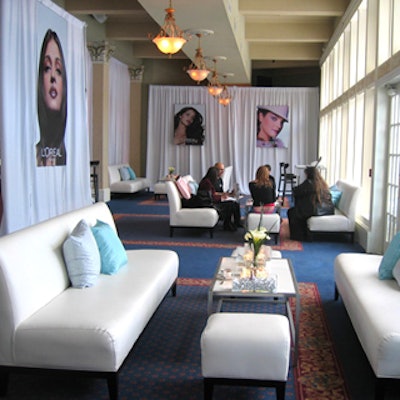The image portrays a spacious living room or potentially a salon, characterized by its predominantly white decor. White curtains adorn the walls, serving as backdrops for various posters of women who resemble models. Prominently, the poster closest to the camera displays the L'Oreal logo. The ceiling features a white-painted beam with four hanging lights, providing illumination to the space. In the foreground, there are empty bench seats adorned with blue and white pillows, along with a white cushioned sofa on the left and another on the right, both accompanied by decorative pillows. A white marble-topped coffee table sits in the center, complementing a blue rug beneath it. In the background, a group of at least five people, including at least one man, are seated on white futons, engaged in conversation. The posters of women in the background are only partially visible, showing them from the head down to the neck, with one model wearing a white hat. Additionally, there is a table with flowers between the chairs, adding a touch of elegance to the setting. On the right side of the image, windows allow natural light to filter into the room.